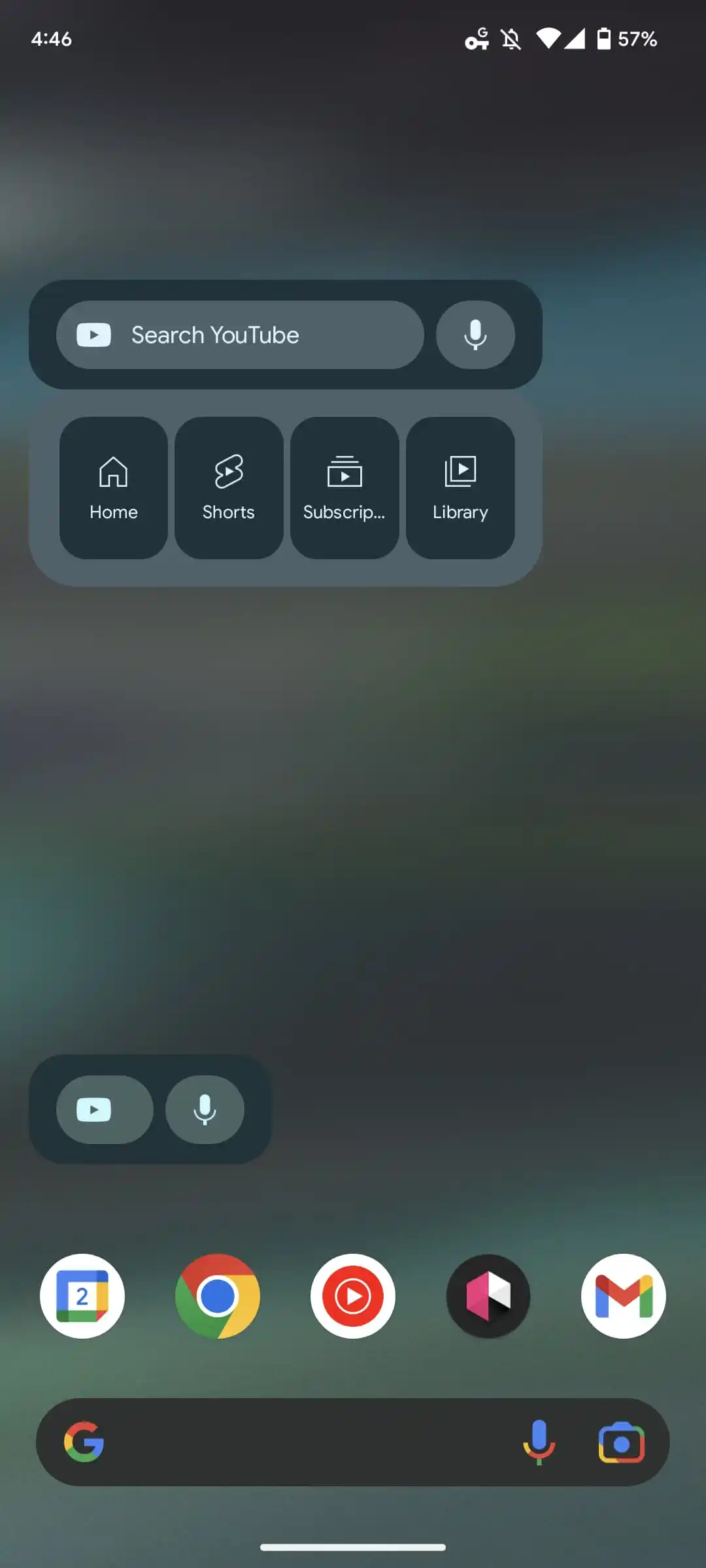The image displays a blurred and out-of-focus background with an abstract gradient. The top part of the background is black, which transitions through shades of blue, brown, green, and purple as it moves downward, eventually fading to gray at the bottom. Overlaying this backdrop is a snapshot of a YouTube app interface on a device with a 4:46 PM timestamp, indicating 57% battery life at the top of the screen.

Prominently featured within the interface is a search bar with the text "Search YouTube" and a microphone icon inside a gray circle. Below the search bar are four black squares labeled "Home," "Shorts," "Subscriptions," and "Library," each paired with corresponding icons above their names. Further down, another area contains a gray circle with a play button icon and another gray circle with a microphone icon.

At the very bottom of the image, there are five icons, including the Google logo, with a Google search bar positioned beneath them. The detailed layout and color transitions create a layered and visually complex representation of the YouTube app interface against an indistinct background.